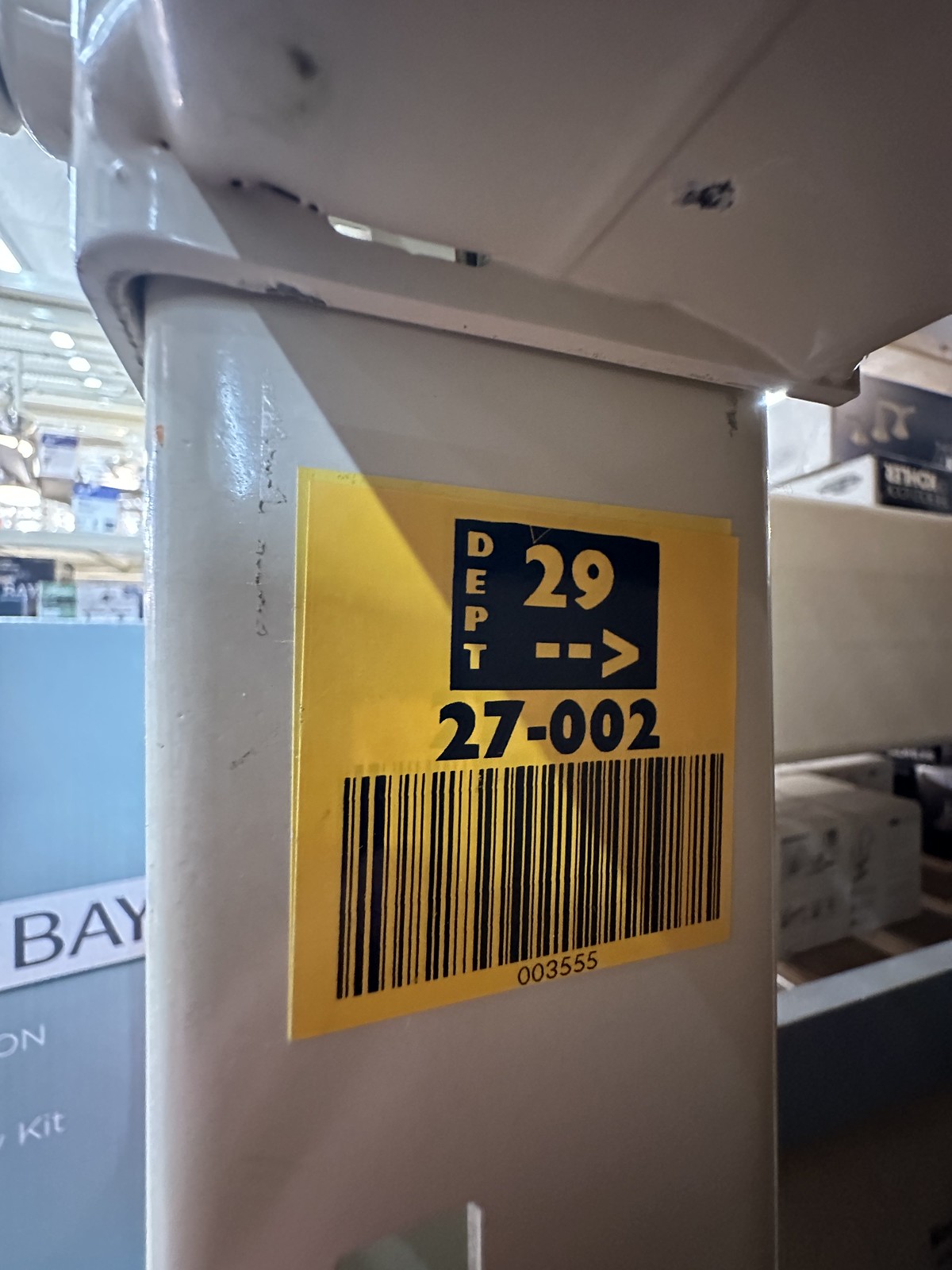This photograph features an intriguing scene captured within a department store. The upper left corner of the image showcases rose and fluorescent lighting that provides a bright and somewhat surreal ambiance to the setting. In the lower left corner, a partially visible sign reads "Bay" and "blue" against a white square set on a light blue background, though the full text of the sign is out of frame and remains unknown.

Much of the focus in this photograph is drawn towards the lower portion, specifically under a shelf where a prominent square yellow sticker is affixed. This sticker features a black box with the text "Department 29" and an arrow pointing to the right, indicating a department direction. Beneath this, the label displays the numbers "27-002" followed by what appears to be a logistic or inventory code "00355". The image captures a mix of utilitarian details and retail aesthetics, providing a glimpse into the behind-the-scenes elements of the store environment.